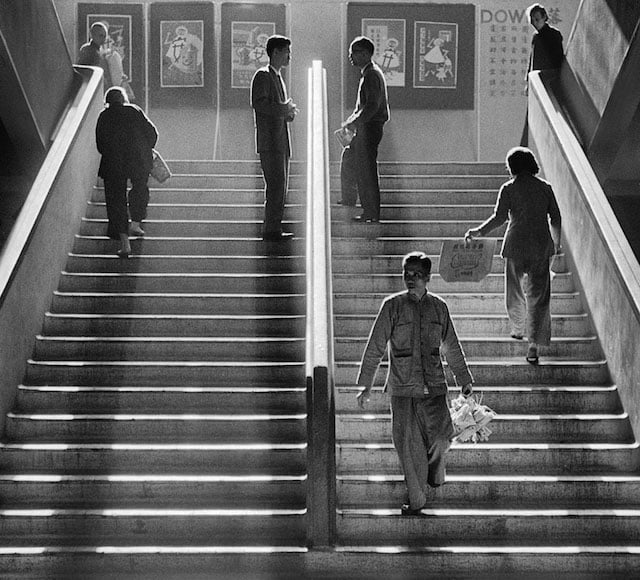The image is a square-shaped black and white photograph, depicting a double set of staircases bustling with activity. This grayscale scene captures seven individuals, seemingly of Asian descent, spread across the staircases. On the left staircase, three people are visible: one person is ascending with their back to us, holding a purse, while another stands at the top watching the ascent. The right staircase hosts four people: a woman is climbing up, a man is descending while facing the viewer, and at the top, another man gazes down the stairs. Between the staircases, two people stand at the top, engaged in conversation.

Behind the staircases, the background features a white wall adorned with black posters, showcasing paintings of stick figures in large dresses. The right side also displays partially obscured text in an Asian script and the prominent letters "D.O.W." or "DAO." Some individuals are carrying bags, and the attire throughout the scene mainly consists of suits or formal wear.

The overall aesthetic, along with the depiction of the individuals and cultural hints, suggests an Asian community center or an old business setting, possibly from the mid to late 1900s. The photograph's gray tones and structured composition evoke a sense of historical and cultural significance within the depicted moment.